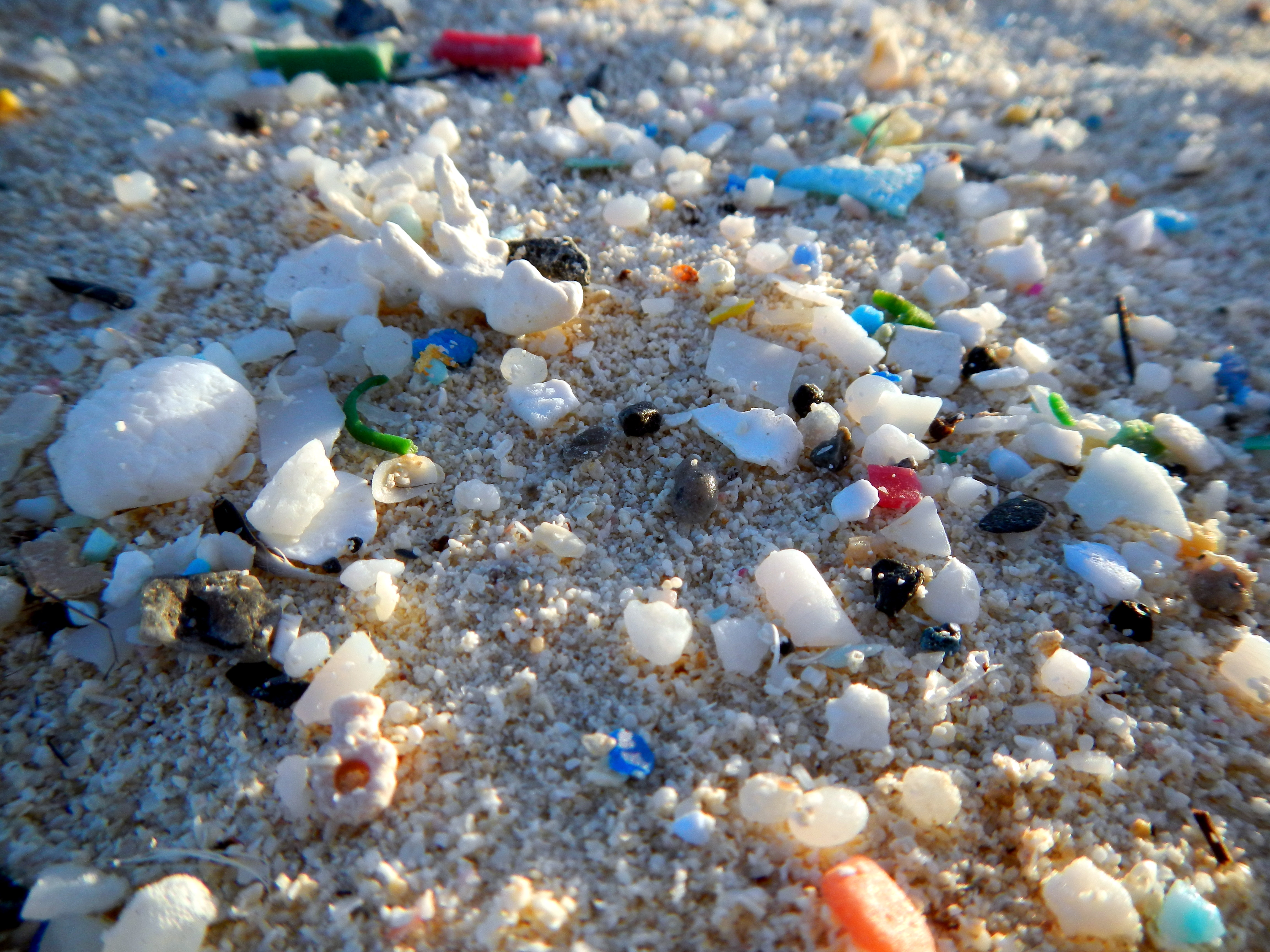The image depicts a vibrant and captivating scene that evokes the visual essence of a beach, yet diverges from the typical sandy shore. The ground is covered with a mix of rocky, granular material rather than traditional smooth sand, creating an intriguing, textured base. Scattered across this rocky ground are a plethora of colorful objects—predominantly white, with splashes of black, orange, and blue. Among these colorful fragments, there are also bits of red and green, adding to the myriad hues.

Closer examination reveals a variety of materials: what appears to be broken seashells mingled with possible pieces of plastic or other debris, and even parts of vegetables like a green pepper segment and a carrot piece. There's sea glass as well, hinted by the smooth, translucent particles glistening in the sunlight. Some of the smaller pieces are indistinct, resembling either tiny rocks and minerals or miscellaneous trinkets. The image becomes less defined near the background, with a noticeable blurriness towards the upper and side edges, suggesting a photograph capturing a moment of ephemeral beauty amidst an unusual yet striking beachscape.